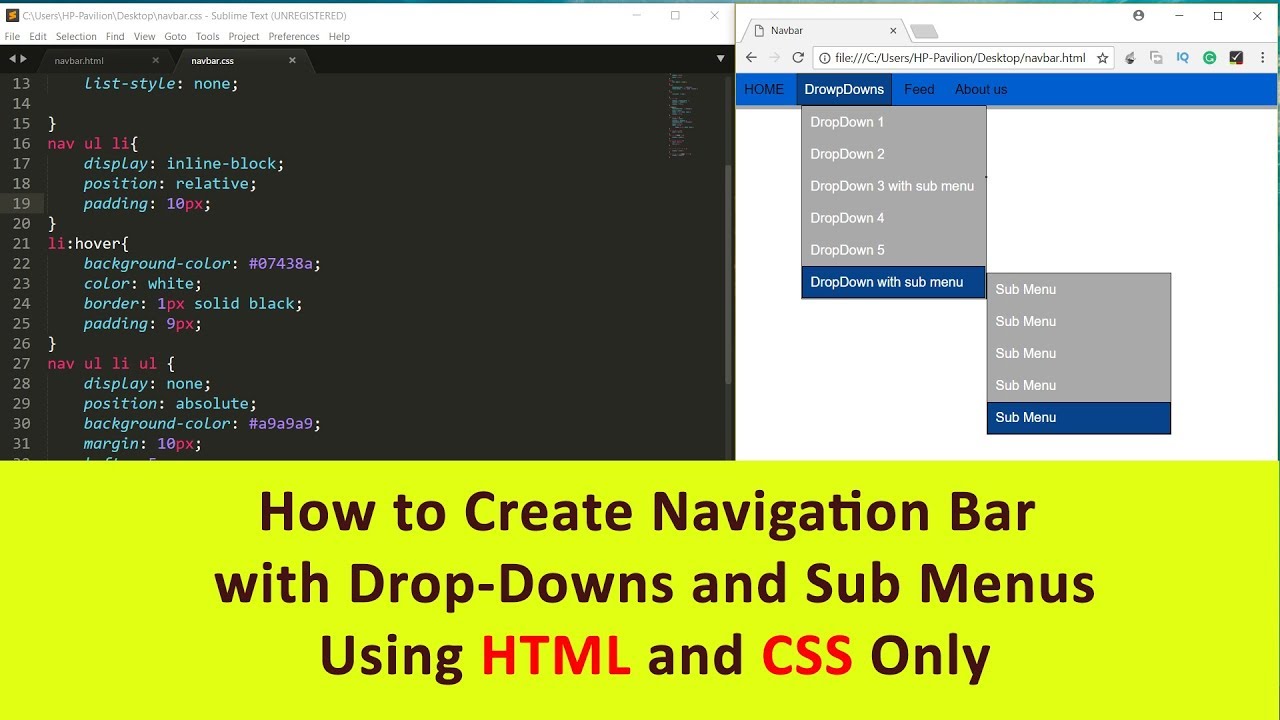The image captures a detailed scene of a coding environment. On the left, a dark gray background displays a dense array of text in a coding editor. The text features various colors: aqua at the top, transitioning into white, red, aqua again, and interspersed with light purple in some areas. Line numbers on the left are uniformly gray except for line 19, which is highlighted with a dark gray rectangle around it. This setup suggests that the user is inspecting an HTML file. 

To the right above, there is a preview of the coded content, showing a miniature version of the interface being developed. At the top of the screen, a white bar features several menu options: File, Edit, Selection, Find, View, Go to, Tools, Project, Preferences, and Help. The title bar reveals the pathway of the open file as "C:\Users\HP\Pavilion\Desktop\navbar.css" and indicates that it is being edited in Sublime Text (Unregistered).

A lime green banner at the bottom stands out with a tutorial title, "How to create navigation bars with dropdown and submenus using HTML and CSS." The terms HTML and CSS are notably highlighted in red, contrasting with the dark purple text of the remaining content.

On the right, another screen displays a different website with a white background. A blue header contains a dropdown menu labeled "Dropdowns." The dropdown menu lists several items: Dropdown One, Dropdown Two, Dropdown Three with Submenu, Dropdown Four, and Dropdown Five, alongside another dropdown item that includes a submenu.

Overall, the image offers a comprehensive view of a coding session, demonstrating the process of creating complex navigation bars with HTML and CSS.